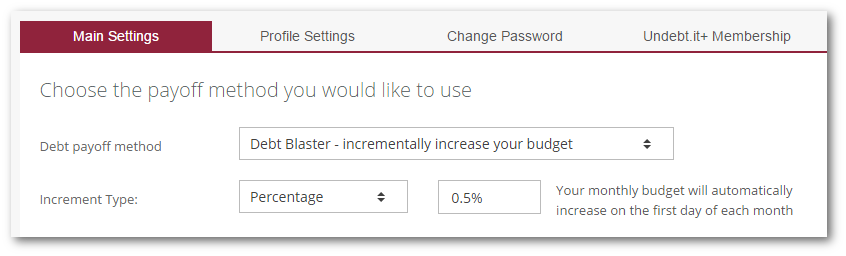The image features a user interface on a white background, highlighting various settings within a financial management platform called UNDEBT.IT. Dominating the interface is a prominent red rectangle, bordered by several white text labels indicating key options such as "Profile Settings" and "Change Password." Additionally, there’s a section dedicated to the UNDEBT.IT Plus membership, which offers users the ability to select a preferred debt payoff method.

Among the options for debt payoff methods is "Debt Blaster," designed to incrementally increase the user's budget. This section is accompanied by an up-and-down arrow icon, symbolizing the adjustable nature of the budget increment. The increment type is set to a percentage value of 0.5%. The interface also notes that the user's monthly budget will be automatically increased by this specified percentage on the first day of each month.